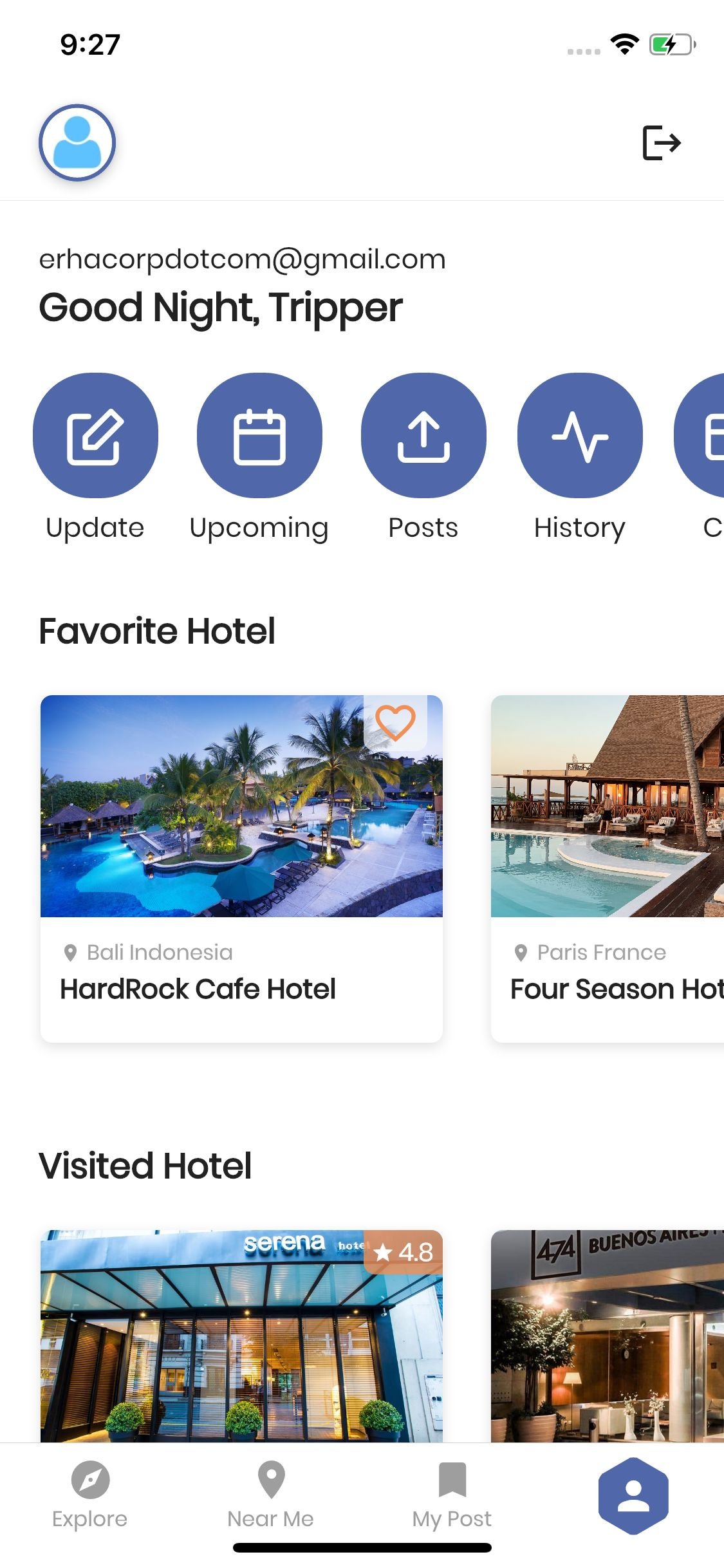**Descriptive Caption:**

The screenshot is from a travel app, showing vital device status and several options for managing travel activities. The current time is displayed as 09:27. The device indicates no cellular service, but a good Wi-Fi connection is available. The battery is at approximately one-third charge and is currently being charged, as indicated by the charging icon.

At the top of the screenshot, there is a blue silhouette icon representing the user profile, followed by an icon that likely signifies the option to log out. The user's email, "erhacorp.com@gmail.com", is visible, accompanied by a greeting "Goodnight, tripper."

Below this, there are distinct headers for navigating different sections: "Update," "Upcoming," "Post," and "History". Under these headers, there is a section titled "Favorite Hotel" featuring images of two resorts: 

1. **Bali, Indonesia, Hard Rock Cafe Hotel** - A poolside resort image marked with an orange heart icon.
2. **Paris, France, Four Seasons Hotels** - Another resort image showcasing a pool and a beautiful sky.

Additionally, there is a section labeled "Visit a Hotel" with two more images:

1. A glass building labeled "Serena" with a review score of 4.8. 
2. "474 Buenos Aires" - However, the full image is cut off, making it difficult to see additional details.

The screenshot offers a snapshot of the app's user interface, highlighting the user's favorite hotels and potential options for upcoming visits.